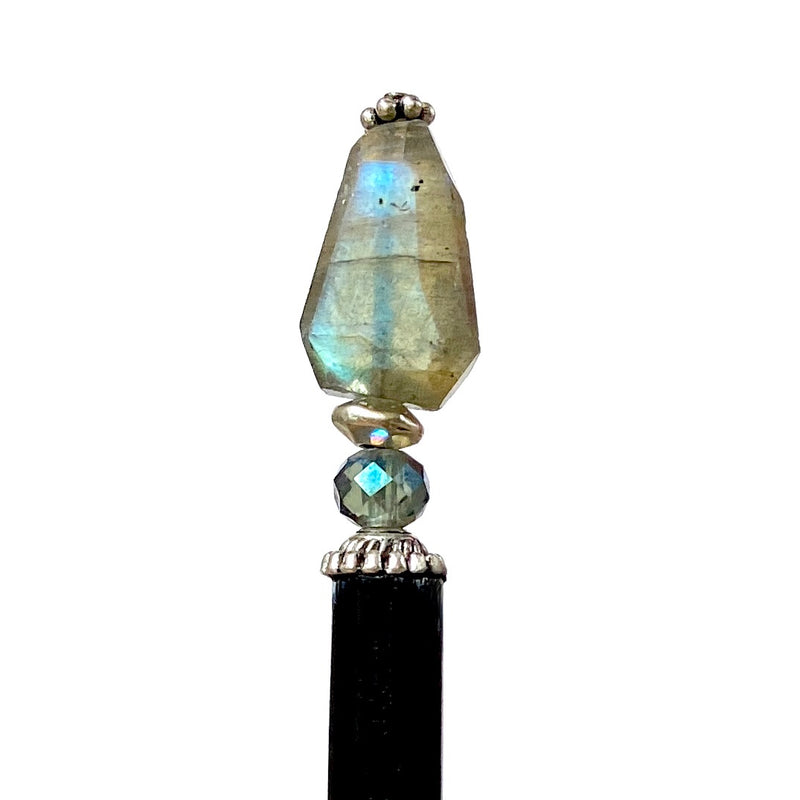This image depicts a unique and intricate decorative piece designed to be an ornament for the top of a black cane. The item boasts an elaborate, antique-looking structure that starts with a shiny black rectangular base. Above the base, the design ascends with a faceted gray bead that glitters under certain light angles. Beyond this bead, there’s an oval-shaped rock in a silver finish, giving off a metallic sheen. Crowning the ornament is a larger, shiny blue rock that reflects light beautifully at various angles. Completing the elegant composition at the top are four small, shiny metal balls arranged in a decorative pattern. The overall look of the piece combines neutral tones with splashes of reflective shimmer, blending elements of both modern and antique aesthetics to create a standout accessory.